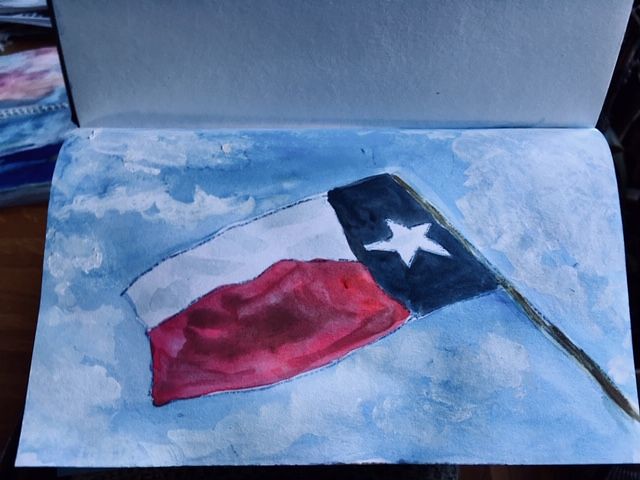The image depicts an open watercolor sketchbook resting on a brown table. The sketchbook is oriented sideways, with the left page positioned at the top and the right page at the bottom. Within the sketchbook, a detailed watercolor painting of the Texas flag is prominently displayed. The flag is composed of a vertical blue stripe with a clear white star on the right side, and horizontal stripes of white and red on the left. Additionally, the flagpole extends from the lower right section of the page. The background of the painting features a blue sky adorned with fluffy white clouds. The overall scene includes other books partially visible around the sketchbook, suggesting it is part of an artist's workspace.